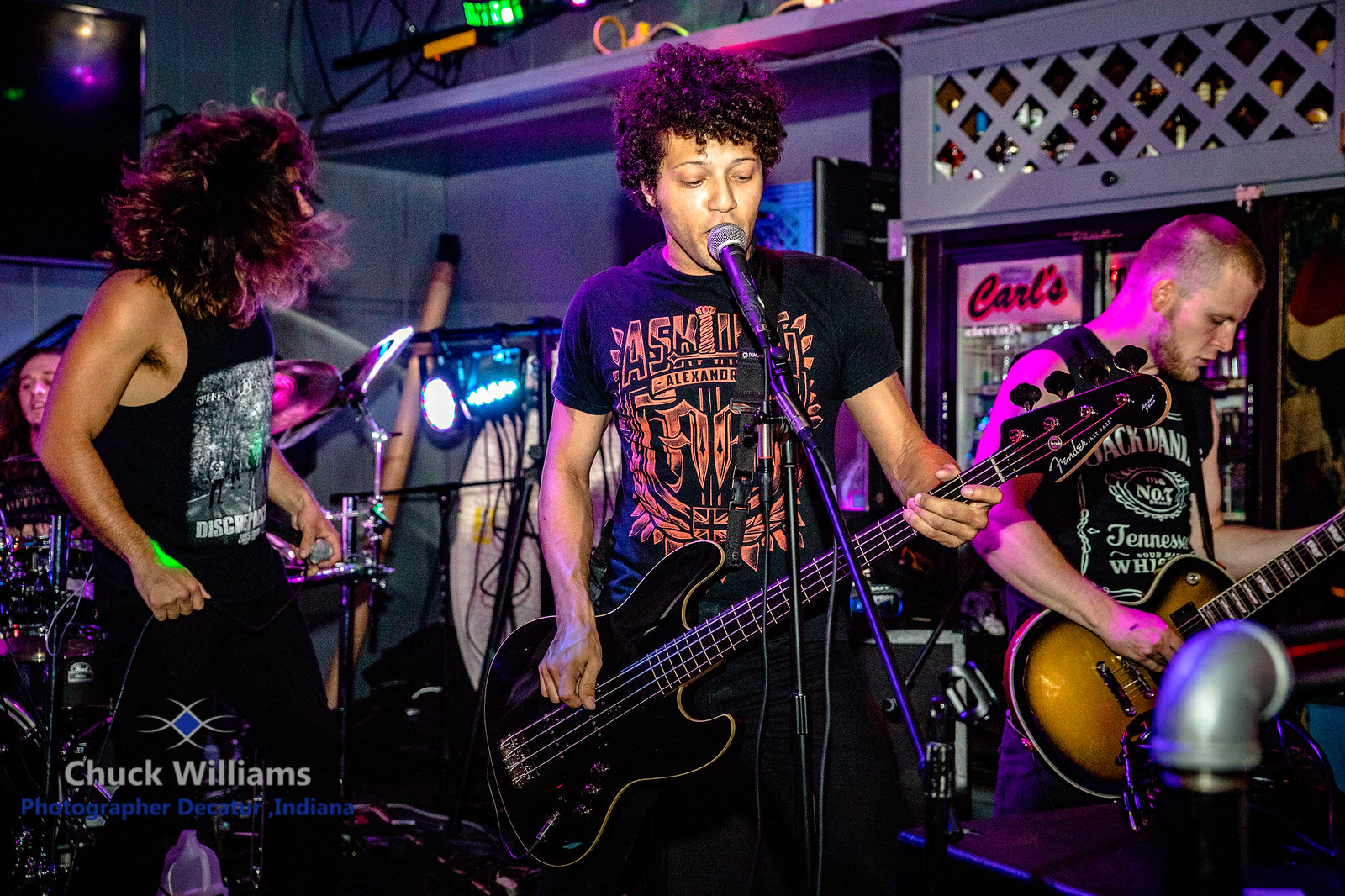The image captures a live performance of a rock band comprised of four male members, donned in black attire, in what appears to be a dark nightclub with gray wooden walls. At the center of the stage is the lead singer with curly hair, singing into a microphone and playing a black guitar. To his left is another man in a black tank top, also playing a guitar, who is intently looking down at his instrument. On the other side of the lead singer is a bald man with a goatee and sideburns, wearing a Jack Daniels t-shirt, holding a black and gold guitar. Behind these three, partially obscured, is the drummer, visible mostly by his face and some of his drum setup. In the background, a sign reading "Carl" and a graded wall can be seen. The stage is predominantly decorated in black, with accents of gray, blue, and white. The lower left corner of the image bears the photographer's credit: "Chuck Williams, Decatur, Indiana."